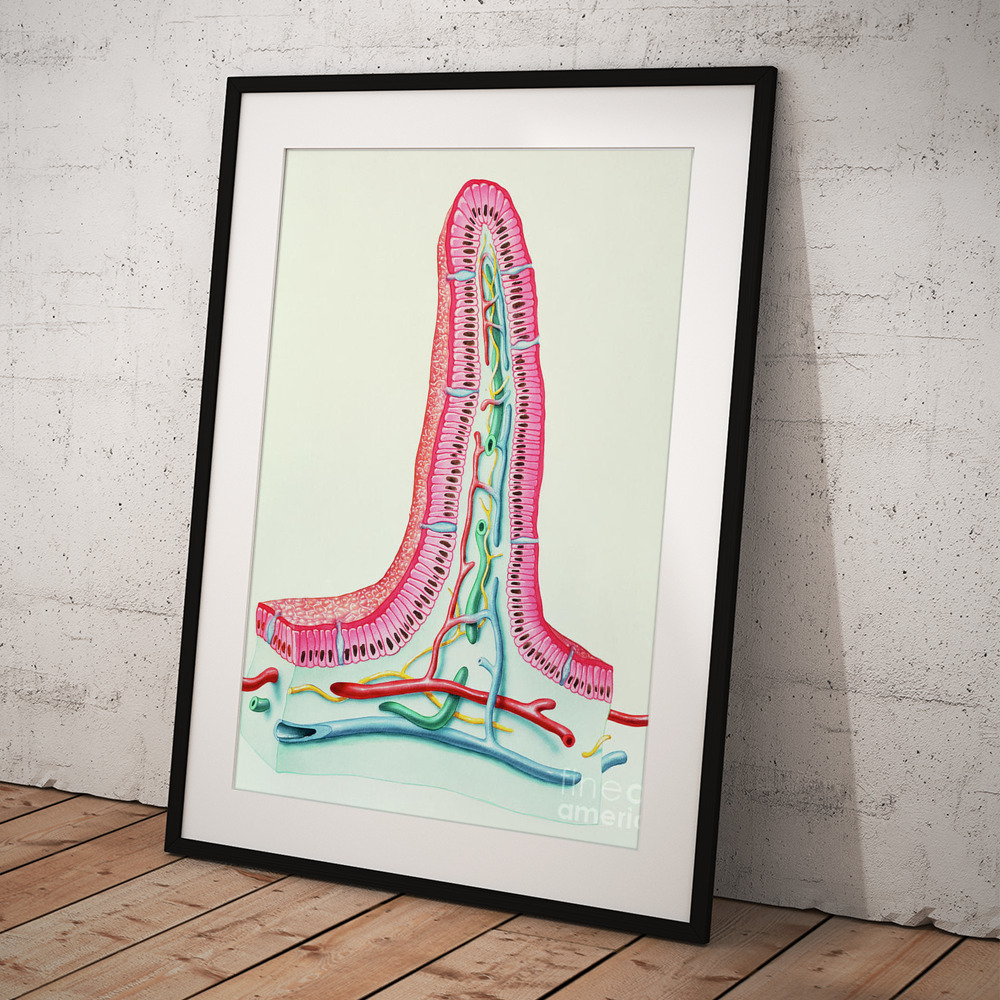A framed print is propped against a natural-looking white stone wall with light brown, unfinished wooden plank floors. The thin black frame encloses a wide white border that surrounds a tall, vividly colored illustration. The image features a faint lime green background and appears to depict a cross-section of a body part, possibly skin. At the top, the artwork shows a red outer layer resembling an outer dermis made of elongated, pink cells that arc sharply upwards. Below this layer, there are intricate, vein-like structures in various colors, including green, yellow, blue, teal, and reddish hues. The detailed depiction, rich in color with highlights of pink, blue, red, and green, suggests a scientific or anatomical focus, capturing the complexity of internal body elements, possibly nerves, arteries, or blood vessels.